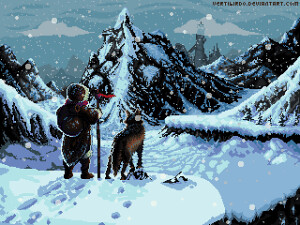The image depicts what appears to be a detailed, computer-generated scene resembling digital art. It captures a snowy, winter landscape where a person and their canine companion stand at the edge of a mountain ledge. The individual, possibly a child or a short adult, is warmly dressed in thick arctic gear, featuring high boots, a long fur coat, and a head covering. They are seen from behind, holding a walking stick adorned with a small red banner. To their right stands a dog, large and wolf-like, possibly a German shepherd or husky, with thick fur and standing slightly above the person's waist. The dog's head is tilted towards the person, as if seeking guidance.

Footsteps in the snow trace a path behind them, indicating their journey to this vantage point. Ahead, snow-covered fir trees stretch into the distance, and an expanse of snow blankets the landscape. Mountains rise in the background, their dark peaks contrasting starkly with the white snow. The sky is blue, filled with clouds from which snow is still falling gently. In the far distance, there appears to be a tower or possibly the remains of a city, although this detail is blurry and somewhat indistinct. Additionally, there is a line of unreadable text in the upper right-hand corner, adding an air of mystery to the scene.